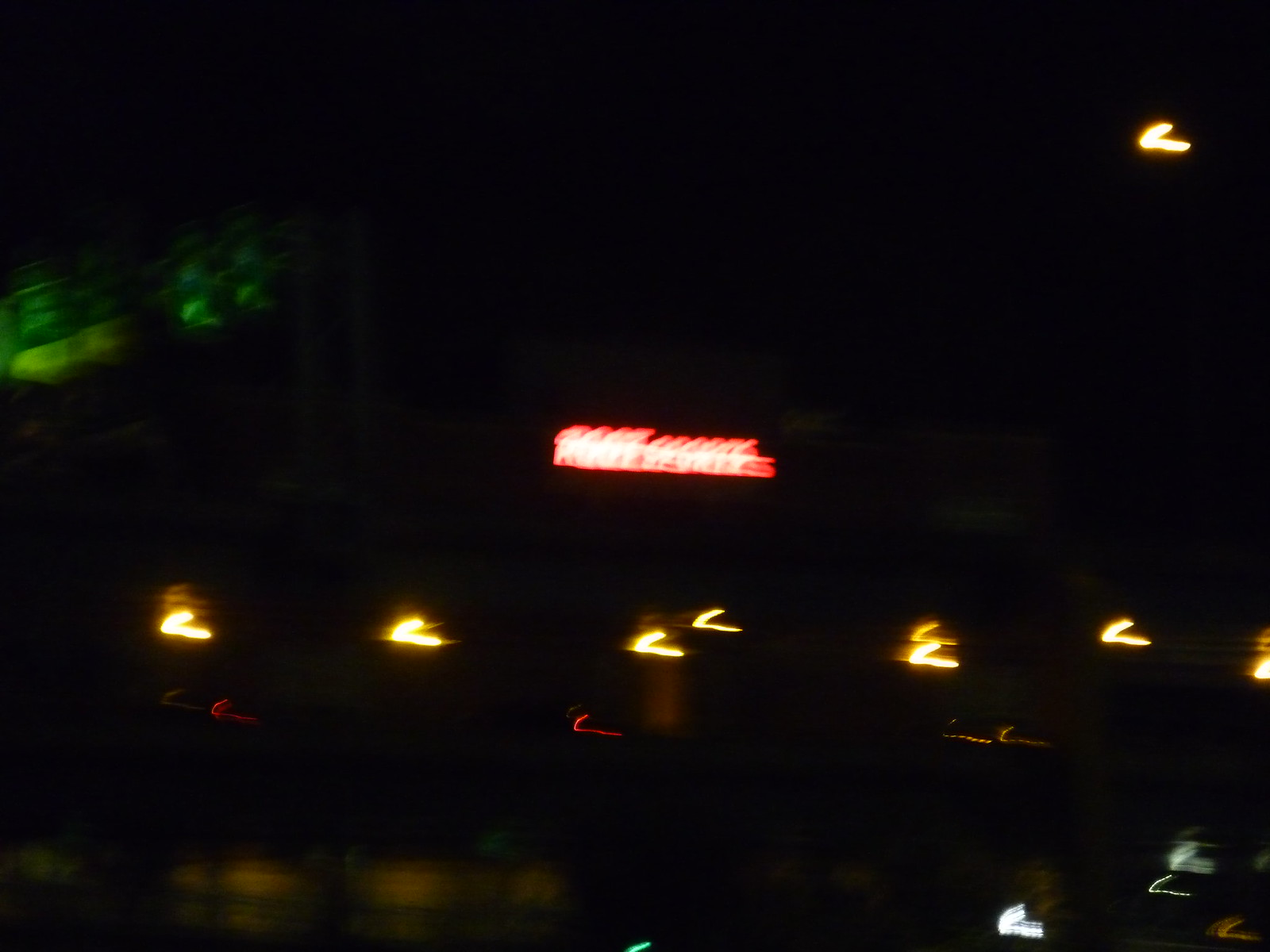The image captures a very blurry night scene dominated by black in both the background and foreground. Scattered neon-like lights punctuate the darkness, their shapes and colors blurred beyond clear recognition. Approximately one-third from the bottom of the horizontal frame, a row of yellowish-white lights forms a sideways V, with the point to the left and the open end facing right. Just below this row, an orangish-red checkmark-shaped light flickers. At the center, a neon sign with white letters on a red-orange background stands out, though its message remains indistinguishable. Towards the upper left corner, a dimly lit upper story of a possible building displays faint green lights, while the upper right corner echoes the V-shaped light motif. The image conveys a sense of motion, perhaps captured from a fast-moving vehicle, and the absence of people, along with the blend of green, yellow, red, white, and blue lights, lends an ambiguous, almost surreal atmosphere to the night scene.